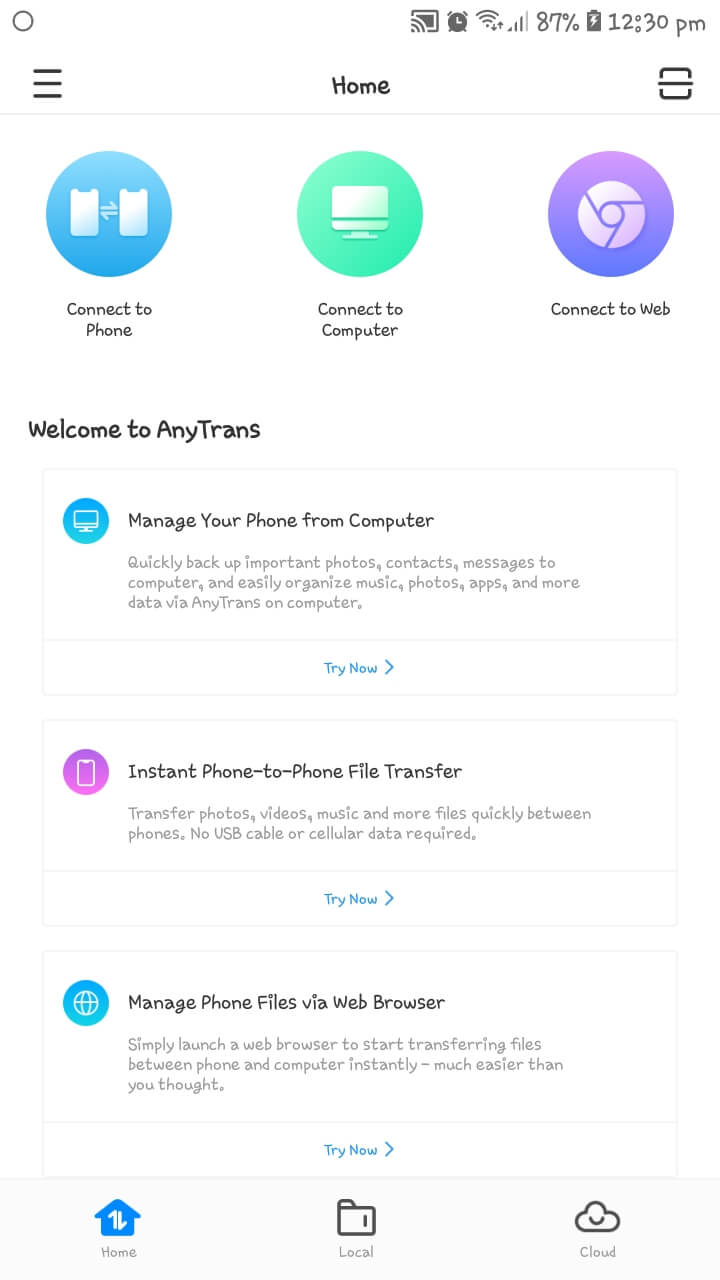This mobile screenshot displays the AnyTrans app home screen. At the top, 'Home' is prominently displayed in the center, with a menu bar icon situated in the top-left corner. Below this, three horizontal icons are clearly visible.

1. To the left, a large blue circle encapsulates two phone images with bi-directional arrows in between, labeled 'Connect to Phone.'
2. In the center, a green circle features an image of a desktop monitor, labeled 'Connect to Computer.'
3. To the right, a chrome icon is displayed within a silver circle nested inside a purple bubble, labeled 'Connect to Web.'

Directly beneath these icons, the text 'Welcome to AnyTrans' is aligned to the left. Below this greeting is a vertical list of options:

1. 'Manage your phone from computer' with a brief description underneath. A blue 'Try Now' button, accompanied by a left-pointing arrow, is centered below.
2. 'Instant phone-to-phone file transfer' followed by another centered 'Try Now' button with a left-pointing arrow.
3. 'Manage phone files via web browser,' again with a 'Try Now' button pointing to the left.

At the bottom of the screenshot, three categories are presented: 'Home,' 'Local,' and 'Cloud,' each with respective icons above the titles. The 'Home' icon is highlighted in blue, indicating the current active page.